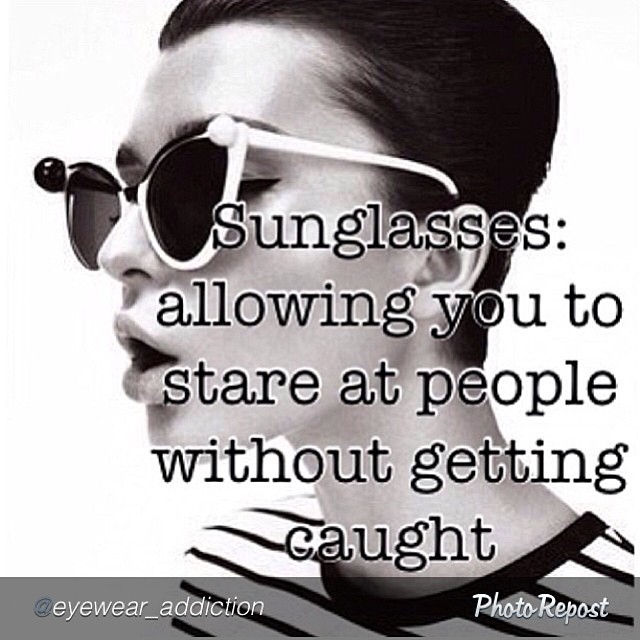This black-and-white profile photograph features a woman with close-cropped black hair and wearing white-rimmed sunglasses with dark lenses. Her mouth is slightly open, and it appears her eyes are closed behind the sunglasses. She is dressed in a high-collared black-and-white striped t-shirt. The image conveys a casual yet striking look, enhanced by an overlay of text which reads: "Sunglasses: Allowing you to stare at people without getting caught." Below this text, in a gray rectangular box at the bottom, is the handle "@eyewear_addiction" with the words "photo repost" on the right-hand side. There is also the presence of a black ball on the left and a white ball on the right side of her sunglasses, adding to the distinctive style of the eyewear.